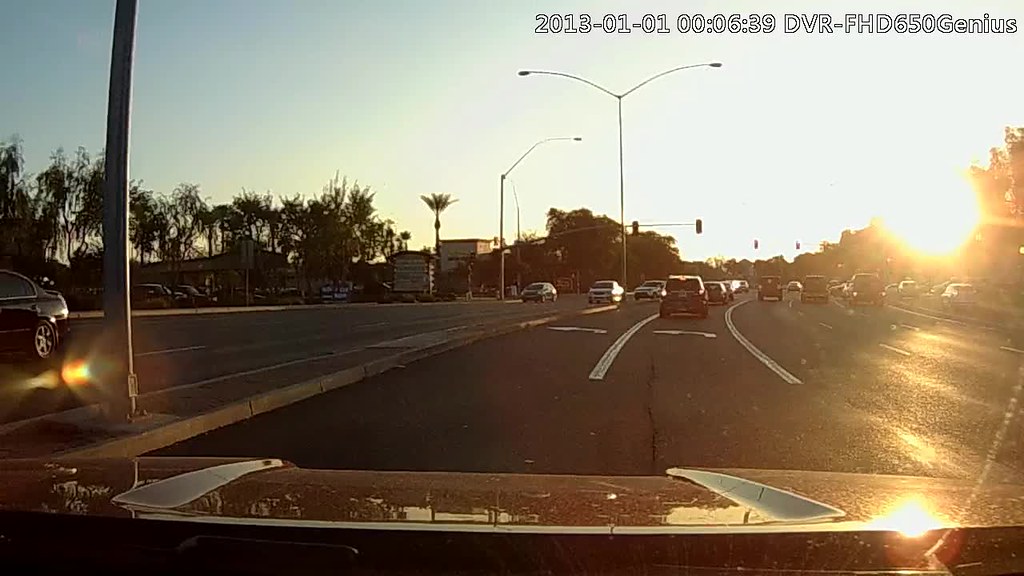This dash cam photo, captured on January 1st, 2013, at 6:39 a.m., shows a car preparing to turn left into the adjacent lane. The early morning light casts a soft glow across the scene, emphasizing the quietness of the first day of the year. On the left side of the image, there is a plaza with a spacious parking lot and several stores. The vehicle, caught mid-turn, appears to be one of the few on the road at this hour, highlighting the stillness of this New Year's morning.